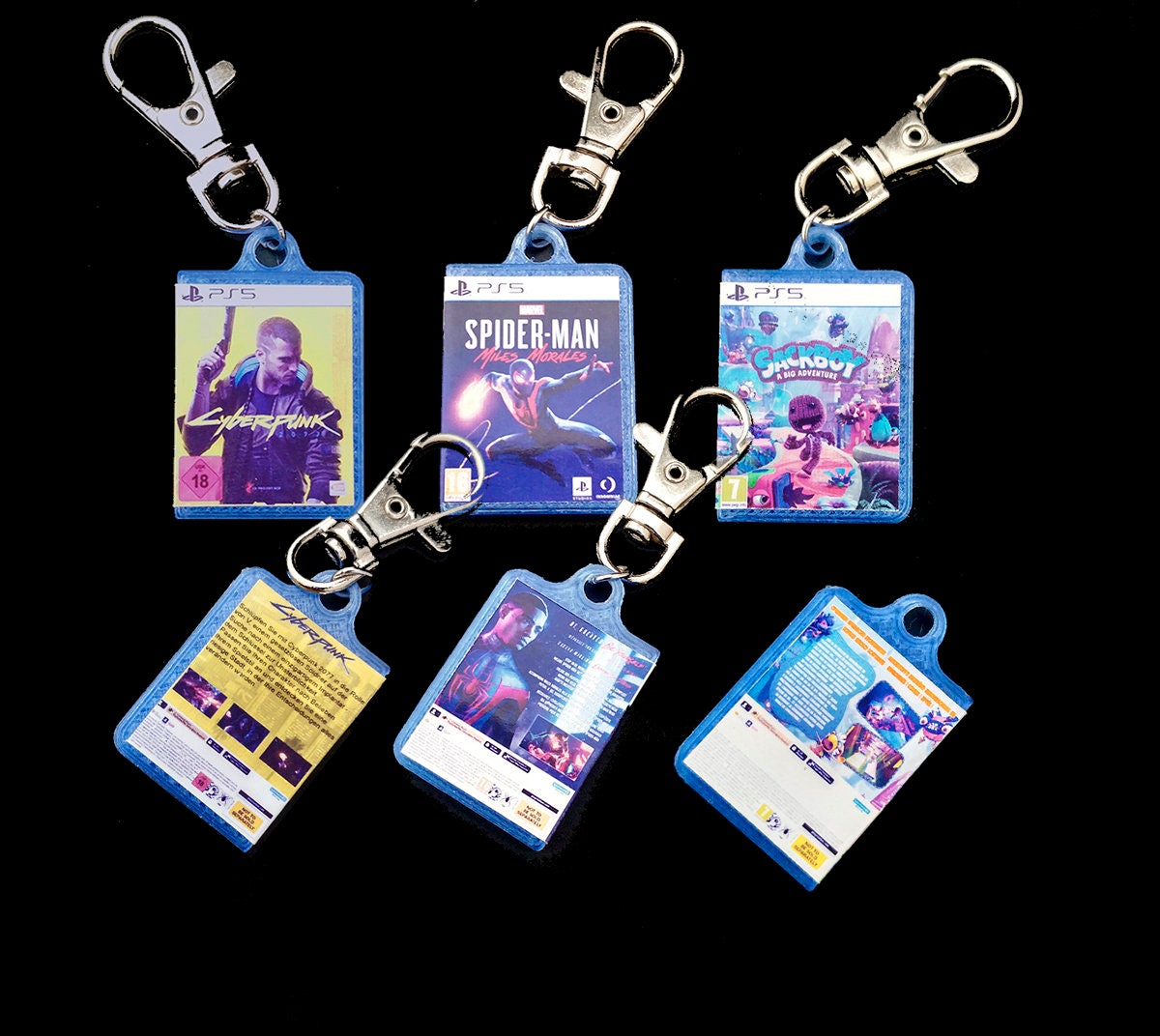Set against a black background, the image showcases six snap-style clasp keychains, arranged in two rows of three. The top row has keychains aligned vertically, while the bottom row has them positioned diagonally from the bottom left to the top right. Each keychain features a square packet hanging from a latch hook, designed to attach to a belt loop. The packets contain cards displaying various PS5 game themes: Cyberpunk, Spider-Man, Miles Morales, and Sackboy: A Big Adventure. The bottom part of the image reveals the reverse sides of these cards, providing additional descriptions of the front images.